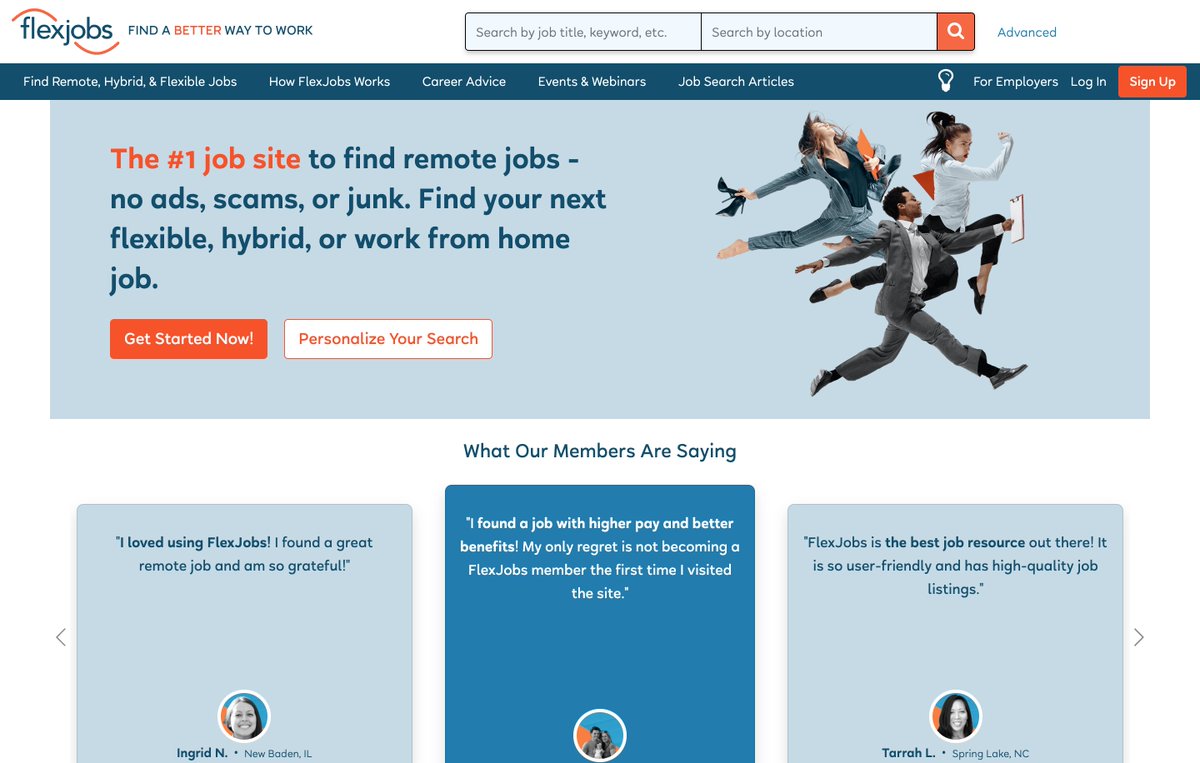The screenshot depicts the homepage of the FlexJobs website, designed primarily for job seekers looking for remote, hybrid, and flexible work opportunities. The background is predominantly white, with a landscape orientation typical for display on a laptop computer or monitor.

**Top Left Corner:**
- The FlexJobs logo features the brand name in lowercase, blue sans-serif font.
- An artistic element is integrated into the logo: a shallow red arch curving over the word "flex" and another shallow red arch under the word "jobs," giving a sense of flexibility and motion.
- Below the logo, in small, all-capital blue letters (with "BETTER" highlighted in red), is the tagline: "FIND A BETTER WAY TO WORK."

**Search Functionality:**
- Adjacent to the logo are two side-by-side search boxes outlined in gray.
  - The left box prompts with "Search by job title, keyword, etc."
  - The right box prompts with "Search by location."
- Between these search boxes, a red square with a white magnifying glass icon serves as the clickable search button.
- Nearby, the word "Advanced" in blue indicates a link for more detailed search options.

**Navigation Bar:**
- A blue horizontal bar spans the width of the webpage, featuring various clickable options in white font:
  - "Find Remote, Hybrid, and Flexible Jobs"
  - "How FlexJobs Works"
  - "Career Advice"
  - "Events and Webinars"
  - "Job Search Articles"
- To the far right, a light bulb icon accompanies the text "For Employers," followed by login options.
- Prominently displayed is a bright scarlet red button reading "Sign Up."

**Promotional Banner:**
- Below the navigation bar, a pale blue and light blue rectangular box extends almost across the page, leaving white margins on either side.
- This box displays an energetic image of three business-casual-dressed individuals, one holding shoes and leaping forward as if dancing.
- Beside the image, text in blue declares: "The #1 job site to find remote jobs. No ads, scams, or junk. Find your next flexible, hybrid, or work-from-home job." The "number one" is emphasized in red with a hashtag symbol.

**Action Buttons:**
- Two prominent buttons are situated beneath the promotional text:
  - A red button with "Get Started Now" in white text.
  - A white button with "Personalize Your Search" in red text.

**Testimonials:**
- Further down, a white bar with the title "What Our Members Are Saying" in blue font spans across the page.
- Below this, three blue squares feature circular user profile photos, along with first names and the initials of their last names, followed by short testimonials about FlexJobs.
- To the right, an open right-arrow icon suggests that additional testimonials can be accessed by scrolling.

This detailed description encapsulates the main elements and features available on the FlexJobs homepage as presented in the screenshot.